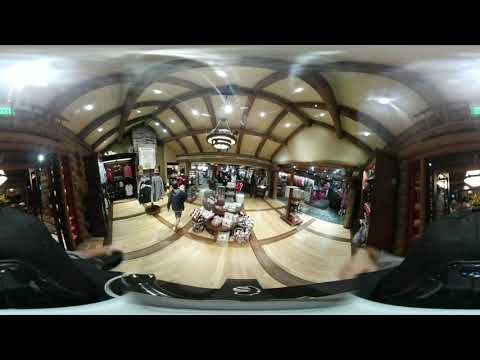The image depicts the interior of a shopping mall with a distinctive curved perspective, giving a warped appearance to all straight lines. A large light fixture hangs prominently from the ceiling, with its reflection visible above. The flooring is tan with a darker wood cross design, emphasizing the pattern. In the center of the scene, directly beneath the light fixture, some merchandise is on display. Shoppers can be seen, with one person in a dark jacket walking through the area. There are stores visible to the right and center, with larger entrances framed in darker wood directly ahead. Store openings and brick walls are discernible amidst hanging clothes and other merchandise displays. The scene is somewhat blurry, but details like wooden ceiling arches and the light's reflection add depth to the setting.